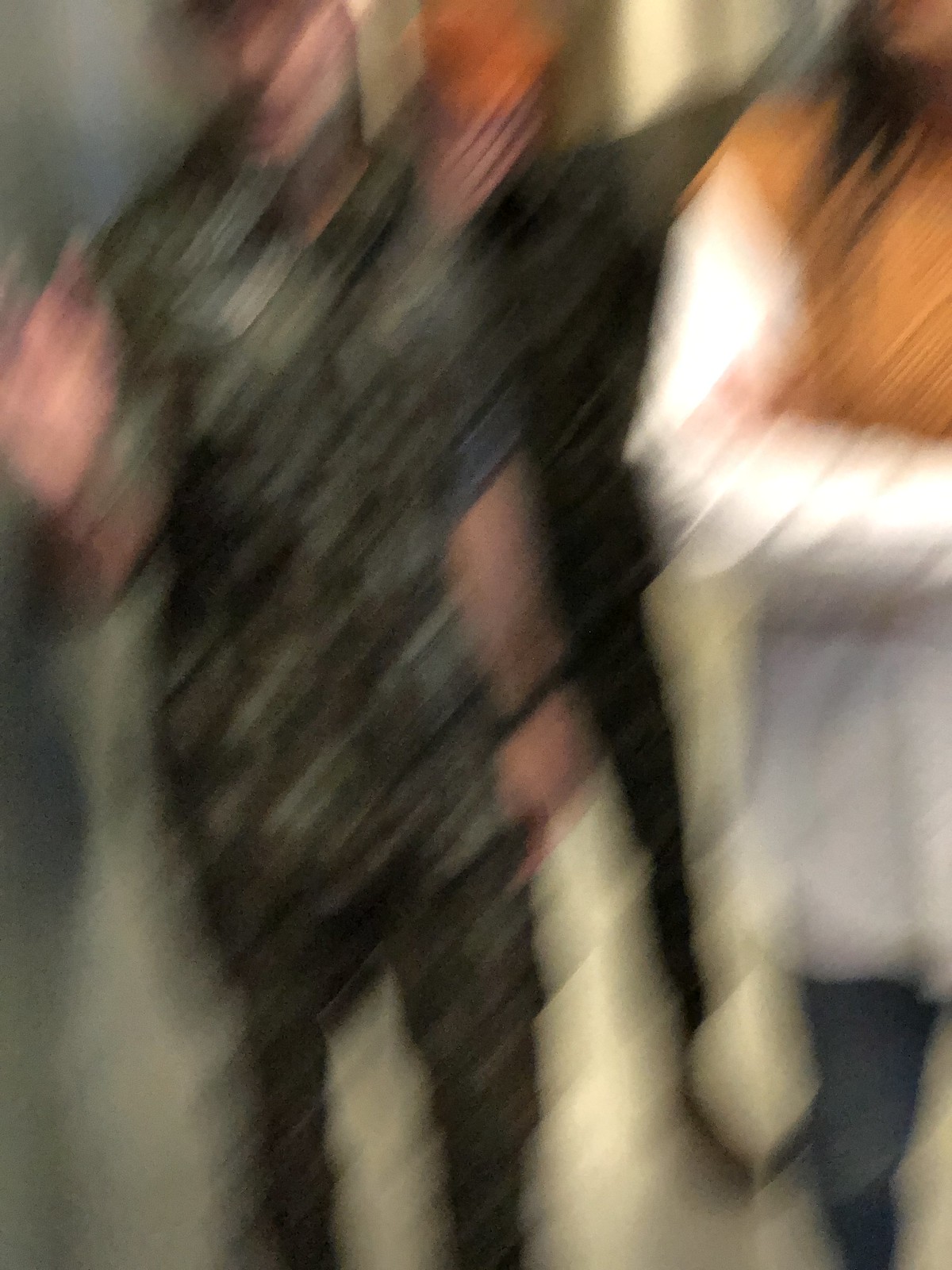This is a very blurry photograph with a grainy, diagonal wave effect, as if the camera was shaken while the picture was taken. The image appears to capture three individuals, although the details are obscured by the blurriness. 

On the left, there is a person who seems to be wearing a camo outfit with bare arms and long pants, raising their right hand. This person might also have a watch on their left wrist. In the middle, towards the background, there's a person dressed in dark clothing with their left arm raised, possibly wearing a black shirt and a black baseball cap. To the right, another individual appears, possibly in a long white shirt or dress, with part of their right arm visible and possibly bent. Some descriptions suggest this person could be heftier, wearing an orange shirt with white sleeves, and possibly having longer black hair or dreadlocks. The tops of all their heads are cut off in the photograph, making their faces hard to distinguish.